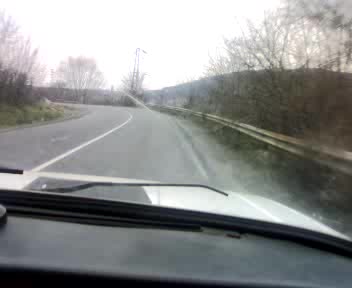This image captures a serene yet striking view from the passenger seat of a vehicle, likely traveling in a right-hand driving country. From this vantage point, you can see the black dashboard and part of the windshield wiper. The vehicle's hood, colored either silver or white with a possible black stripe down the middle, peeks into the frame. The black asphalt road winds to the left, bordered on the right by a sturdy guardrail that hugs the edge of a steep, mountainous cliff.

The right side of the image displays the rugged shoulder of the road, interspersed with sparse wintertime trees and patches of green undergrowth. These trees also frame the scene on the left and straight ahead, accentuating the road’s sharp curve. Beyond the immediate foreground, the landscape opens to a vast valley, leading the eye to a distant mountain shrouded in the muted tones of a white winter sky. The stark colors of black, white, and gray dominate the image, crafting a minimalistic yet captivating winter tableau.